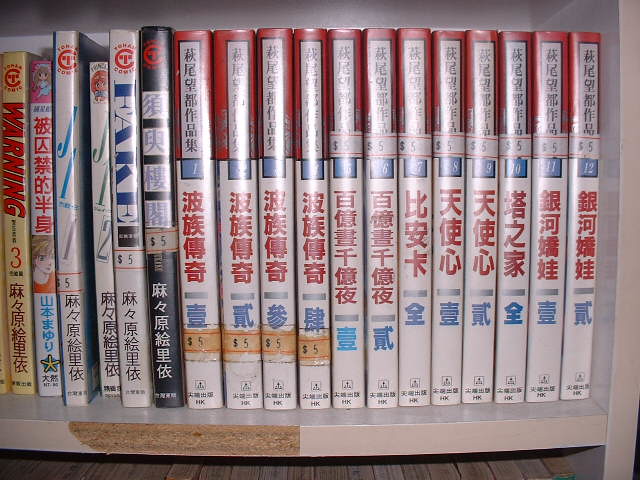The photograph features a bookshelf densely packed with around 15 neatly arranged books, primarily in Japanese or Korean. Most of the books belong to the same series, characterized by their distinctive red and white coloring: the top portion of the spine is red, while the lower portion is white, each adorned with black and red symbols. A notable feature within these books is a blue square marked with the number 12. Several of these books have price tags indicating $5. The last few books on the right side differ; one has a yellow spine with the word "warning," and another features the term "fake," along with various others, some including anime characters, hinting they might be manga. The bookshelf itself is made of inexpensive white material, visibly chipped at the bottom left to reveal particle board. The scene is set against a wooden floor, suggesting the bookshelf is situated at ground level.